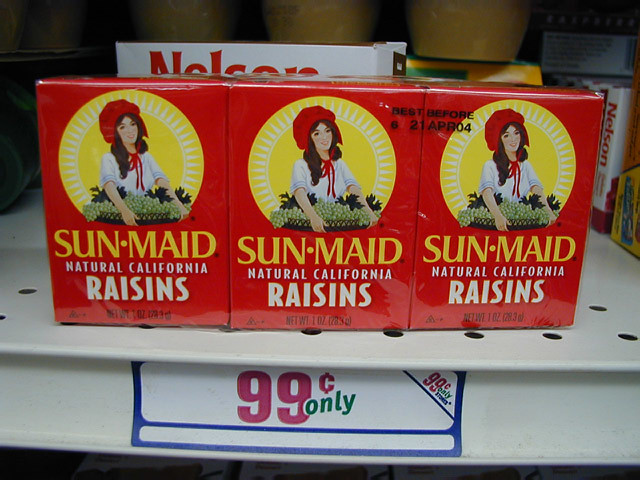This detailed photograph illustrates a close-up view of a grocery store shelf displaying a three-pack of Sun-Maid Natural California Raisins, prominently featured at the edge of the white metal shelf. The product consists of three small, red boxes, each emblazoned with yellow and white text. The logo is a bold yellow sun with radiating white rays, set behind an illustration of a woman with brown hair. She wears a red bonnet tied around her neck and a white blouse, and holds a large tray of green grapes. The text on the packaging reads "Sun-Maid" in yellow, followed by "Natural California" and "Raisins" in white. The total weight and a "Best Before" date of April 21st, '04 are also visible. Below the raisins, affixed to the white trim of the shelf, is a price tag with a blue border. Inside, it reads "99¢ only," with "99¢" in red and "only" in green. The shelf features standard holes and another glimpse of various products scattered behind the raisin pack, suggesting it might be among the last available of its kind.